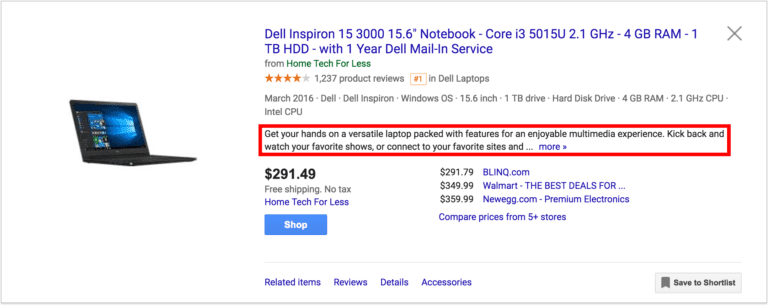**Detailed Caption:**

Discover the Dell Inspiron 15, a reliable and feature-packed laptop perfect for home or work. Priced at $291.49 with free shipping and no tax from Home Tech For Less, this 15.6-inch notebook is powered by an Intel Core i3-55015U processor at 2.1 GHz. It comes with 4 GB of RAM and a spacious 1 TB HDD, ensuring ample storage and efficient performance for everyday tasks.

Highlighted by a red box in the image, the promotional text reads: “Get your hands on a versatile laptop packed with features for an enjoyable multimedia experience. Kick back and watch your favorite show or connect with your favorite sites and more…” Accompanied by a blue right arrow, this detail emphasizes the laptop’s multimedia capabilities.

Rated 4 out of 5 stars based on 1,237 product reviews, the Dell Inspiron 15 is highly recommended and ranks number one in Dell laptops. 

Additionally, the product is available through alternative sellers, with prices listed at $291.79 on BLINQ.com, $349.99 at Walmart, and $359.99 at Newegg. This demonstrates the competitive pricing and options available to consumers seeking the best deal.

This laptop also includes a one-year mail-in service warranty from Dell, offering peace of mind with your purchase. Compare prices from over five stores to ensure you get the best offer on this quality device.